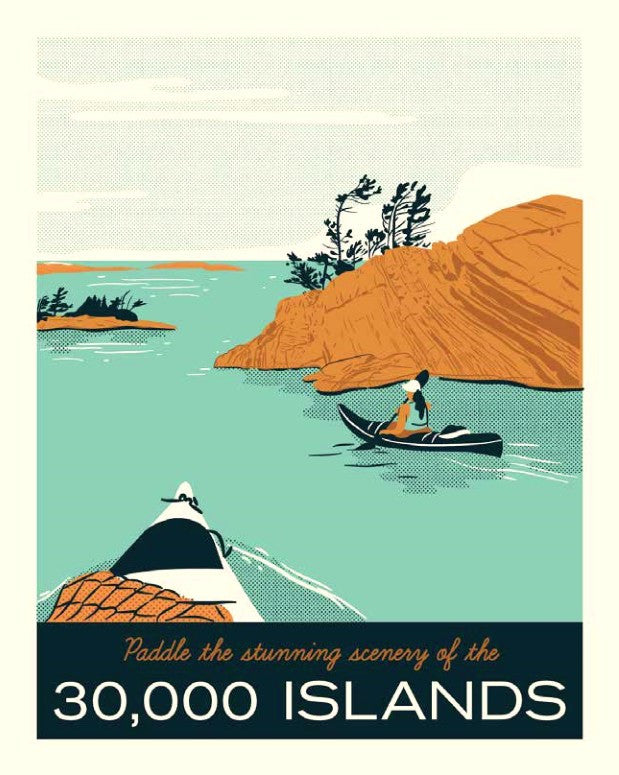This cartoony tourist poster, set against a grey sky with white clouds, invites you to "Paddle the stunning scenery of the 30,000 islands," as stated in a sophisticated font across a black banner at the bottom of the image. The banner features "30,000 islands" in bold white letters, while the rest of the text is in orange. The main scene showcases tranquil, green-blue waters dotted with four small islands, some adorned with dark trees or bushes. A woman with long black hair wearing a white hat and a blue life jacket paddles a black kayak. The image, which seems to be viewed from another kayak, includes just the nose of this second boat in the foreground, evoking a sense of immersive adventure. The islands appear rocky with brown shrubbery, completing the idyllic and inviting landscape intended to transport viewers to this serene locale.